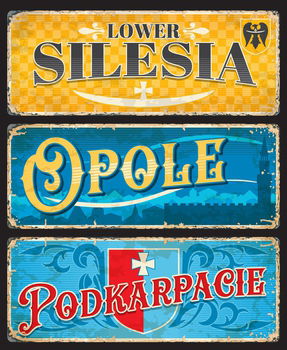The image showcases three decorative, early 1900s-style rectangular signs stacked vertically, each surrounded by a thin white rim and set against a black background. The top sign is a yellow checkered pattern, featuring the text "Lower Silesia" in black lettering, adorned with white fleur-de-lis designs on either side of "Lower" and a white cross and curved smile shape below "Silesia." A black eagle on a crest is positioned in the upper right corner of this sign. The middle sign displays a blue-toned, simplistic silhouette of a city skyline, likely London, with a darker blue depiction of a structure resembling Big Ben on the right and the text "Opole" in yellow. The bottom sign has a bright teal background with a centrally located red and blue crest bearing a white cross, and the text "Podkarpacie" in red.